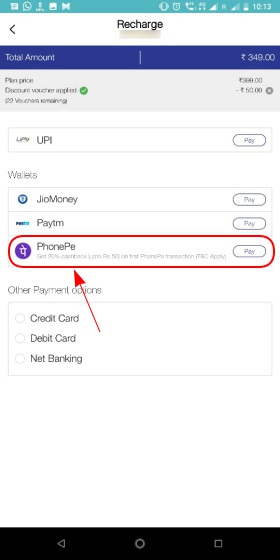This image, captured from a smartphone screen, illustrates a recharge transaction interface. At the top, a prominent "Recharge" header is displayed. Below this, there is a blue background section showcasing the total amount labeled "349 Rupees." The text immediately beneath this amount is blurred and not legible due to its small size.

Further down, the payment method "UPI" is indicated, along with various wallet options like "GinoMani," "PayTM," and "PhonePe." The "PhonePe" option is highlighted with a red outline, possibly showing it as the selected method. An arrow pointing downwards emphasizes this choice. Beside the wallets, there’s an option to "Add a payment option," listing possible methods like credit card, debit card, and net banking, each accompanied by a checkbox.

On the right side of the screen, 'Pay' buttons are aligned with each payment option—UPI, wallets, credit card, debit card, and net banking. The background of the entire screen is white, providing a stark contrast to the blue background highlighting the total amount.